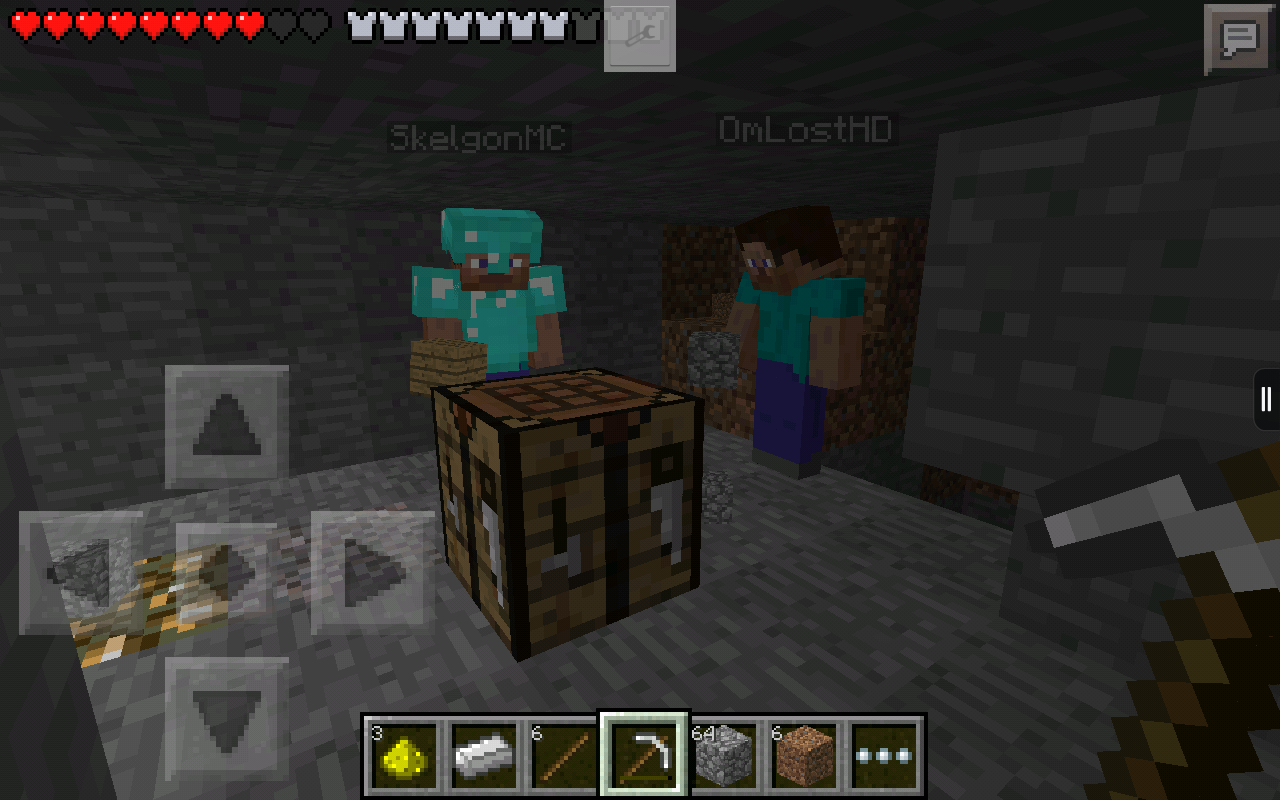This detailed landscape-style Minecraft screenshot showcases a small 3x3 room with grey rock walls, ceiling, and floor. In the center of the room is a crafting table atop a solid grey rock surface. The composition features a person observing two Minecraft players: one on the left, named SkelgonMC, adorned in diamond armor with a diamond helmet and holding a brown block, and the other on the right, named OmlostHD, dressed in a teal blue shirt, dark blue denim jeans, and grey pants with a grey rock in hand, wearing no armor. Both player names appear in light grey text against a black background above their characters.

In the inventory menu displayed, items include yellow powder dust, an iron bar, six straight rods, a silver or iron pickaxe, 64 cobblestone blocks, and six dirt blocks. The player's health status is indicated by the hearts in the upper left corner, showing only two hearts missing, and the armor status, with three plates missing. Surrounding the inventory items at the bottom is a diagram featuring gold, a white object, a brown rod, a brown axe, a grey cube, a brown cube, and three white dots. On the bottom left of the screen, directional arrows point up, down, left, and right, with a diamond-shaped icon in the center, complementing the in-game HUD elements.